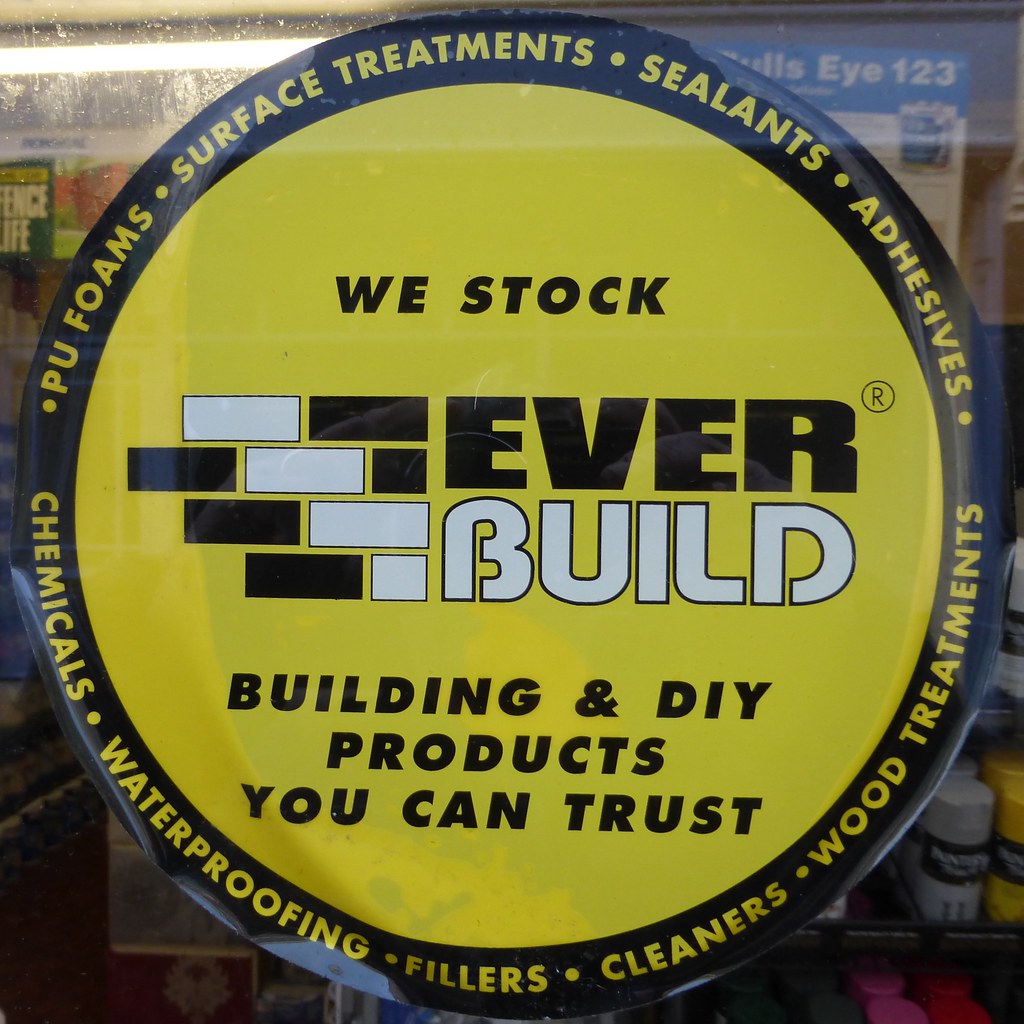The photo showcases a vibrant, circular sign prominently displayed at the center of a glass window, possibly situated in a dimly lit hardware store. The sign features a striking black border with bold yellow text that advertises various products: "PU Foams, Surface Treatments, Sealants, Adhesives, Chemicals, Waterproofing, Fillers, Cleaners, Wood Treatments." Dominating the yellow core of the sign is a prominent "We Stock EverBuild" slogan, with "Ever" in black text, "Build" in white text, accompanied by a logo with black and white brick illustrations. Beneath this, in smaller black text, it reads, "Building and DIY Products You Can Trust." Through the window, faint outlines of hardware store items such as spray paint cans in colors like white, yellow, gray, pink, and red, are visible, adding context to the setting. The detailed sign and the partially visible store interiors together paint a vivid picture of a robust hardware supply environment.